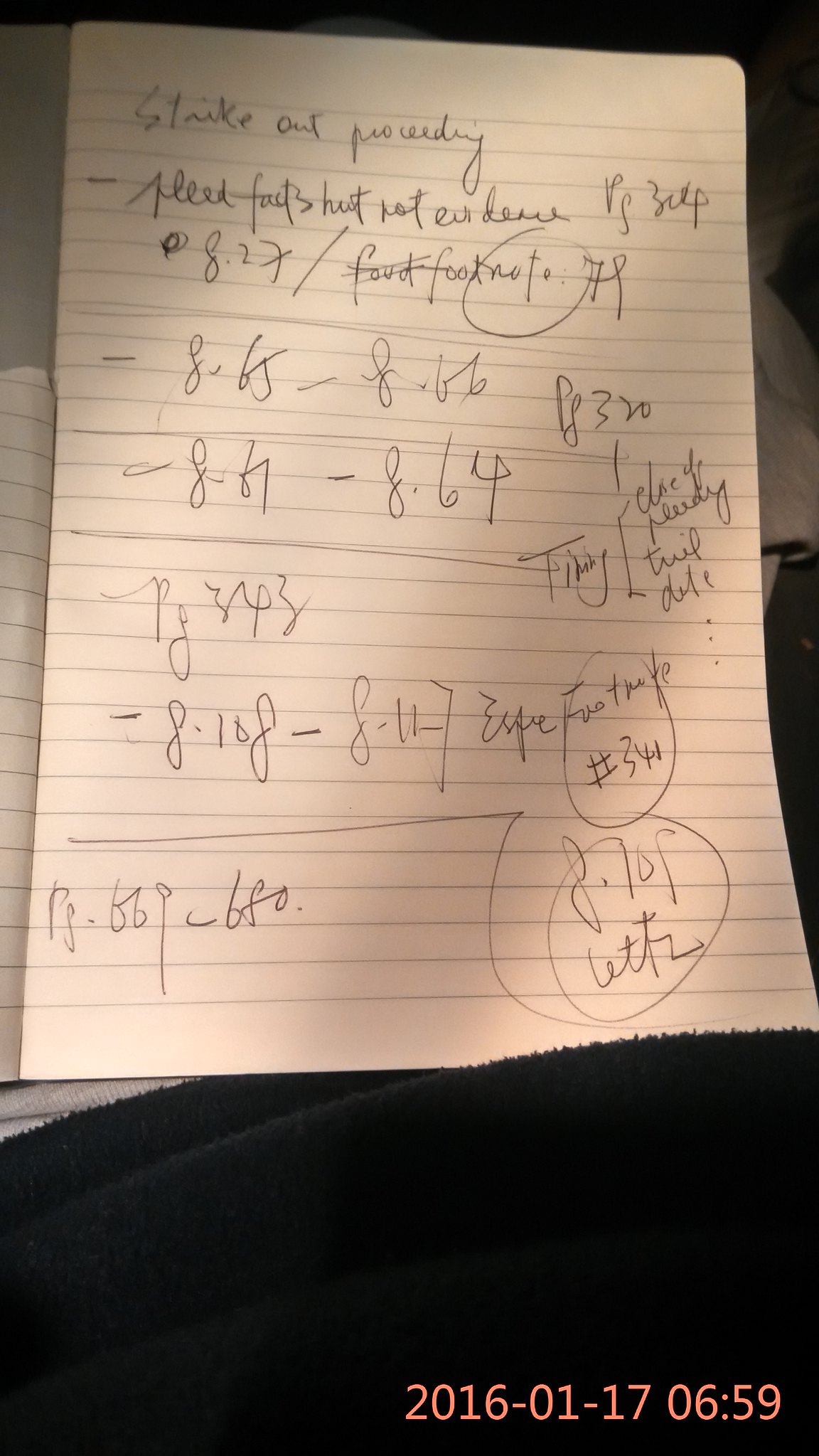This photograph captures a sheet of lined paper set against a black background, with additional lined papers partially visible behind it. At the bottom of the image, there is a timestamp in a pinkish-orange hue that reads "2016-01-17 06:59." 

The sheet features handwritten notes and equations in black ink. At the top, the phrase "stake out proceeding" is written in cursive. Below this, several equations and notes are visible, though they are somewhat difficult to decipher. The text begins with "feed facts best not evidence pp," followed by "8.27 divided by footnote 7r." Below this equation, a hastily drawn line separates it from another set of calculations, "negative 8.6 minus 8.66," which appears adjacent to the page number "320."

The page references five sets of footnotes, suggesting that these notes are related to a book. The document has an overall hurried and informal appearance, adding to the sense of personal annotation or rapid jotting of thoughts.